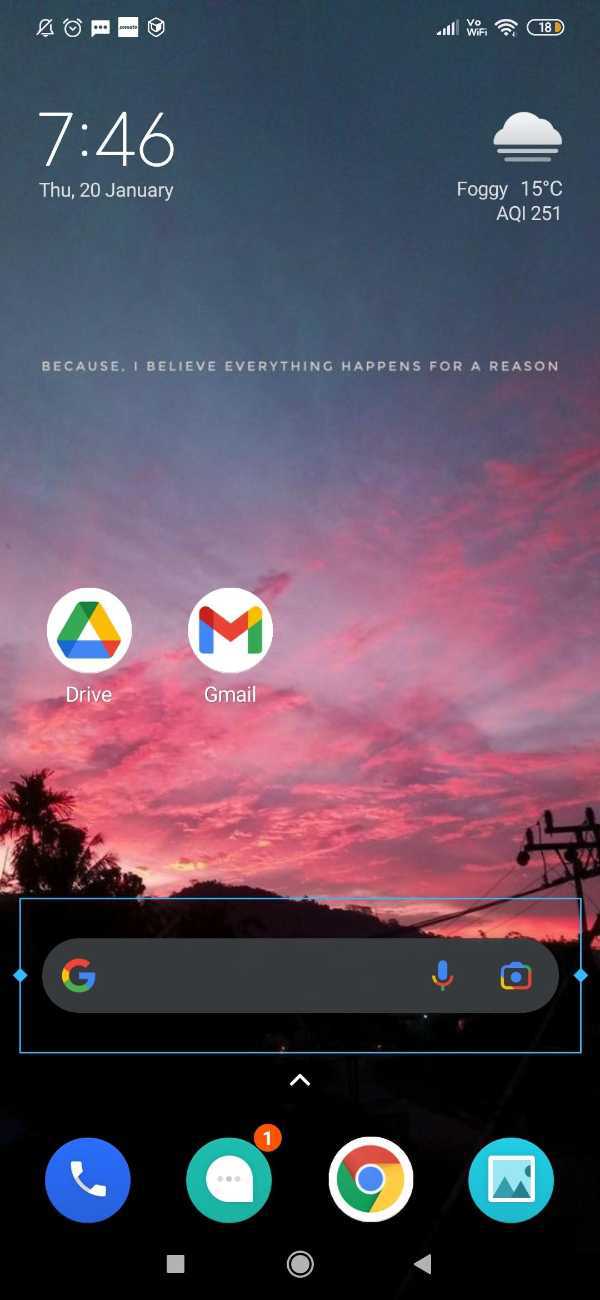This screenshot of a mobile device's screen provides a plethora of detailed information. At the top of the screen, an alarm icon is visible, alongside additional icons indicating ongoing conversations and notifications, which have been silenced, depicted by a bell with a line through it. The carrier signal is strong with four bars, and Wi-Fi is enabled. A battery icon shows a low battery life at approximately 18%. The current time is 7:46 AM on Thursday, January 20th. The weather is foggy, with a temperature of 15°C, illustrated by a cloud icon.

The wallpaper of the device is a visually captivating gradient of pink, blue, and purple hues reminiscent of a sunset, accentuated by the silhouettes of palm trees and a darker foreground at the bottom. An inspiring quote reads, "Because I believe everything happens for a reason," featured prominently over the background. The home screen includes two notable app icons: Google Drive and Google Gmail. Additionally, a Google search bar is present at the bottom, complete with the Google logo, a microphone icon for voice searches, and a camera icon for visual searches.